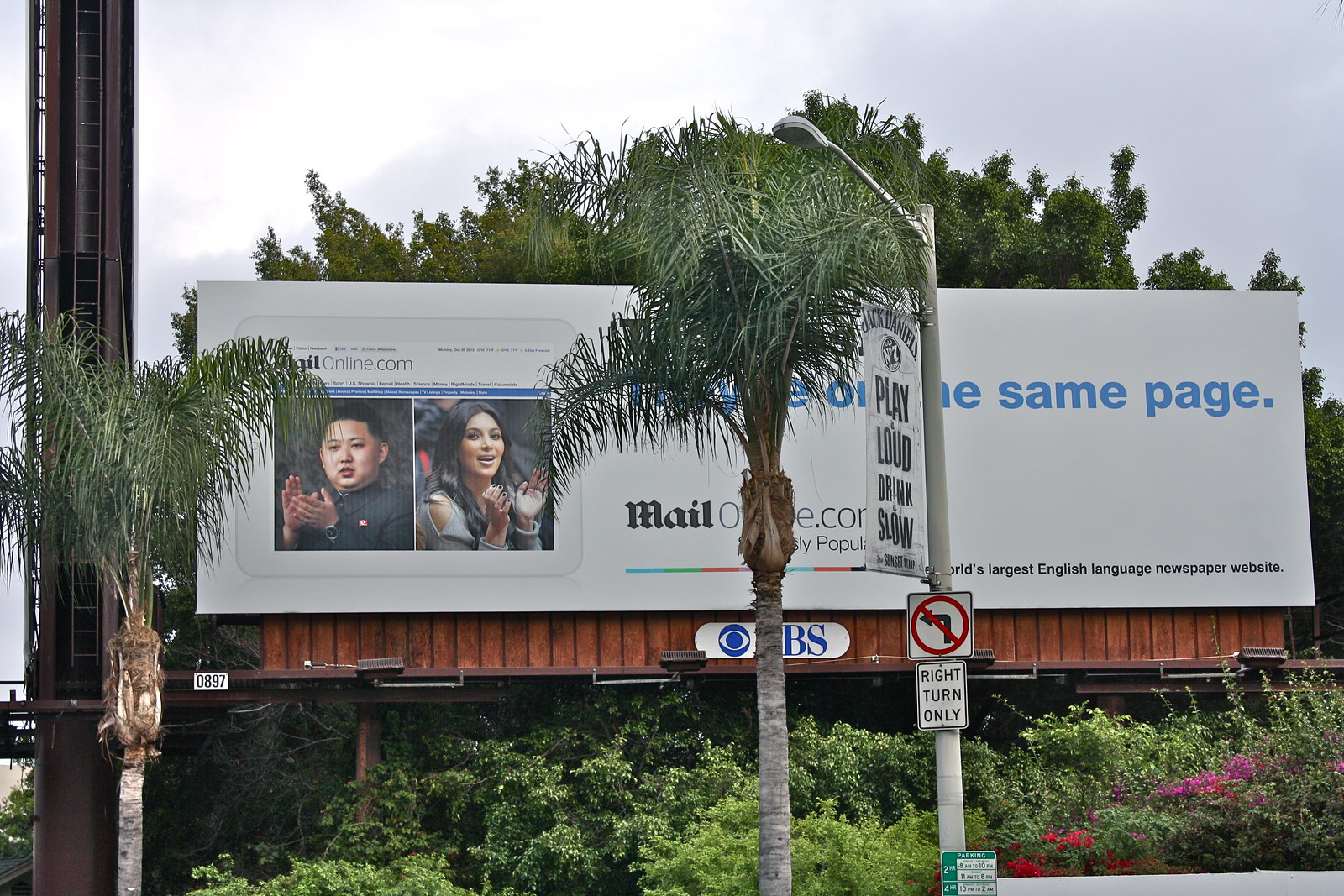The image depicts a large white billboard for MailOnline.com, recognized as the world's largest English language newspaper website. The billboard features a divided image showing Kim Jong-un, the leader of North Korea, clapping on the left side, and the media personality Kim Kardashian clapping on the right. The headline includes partially obscured blue text that presumably includes the phrase "same page." The billboard, set against a tropical backdrop with tall palm trees and a large streetlight obstructing part of the view, also has a smaller sign hanging from the streetlight advertising "Chuck Daniels play loud drink slow" and a right turn only sign directly below it. The word CBS is visible at the bottom of the billboard. The scene is captured during the day, with clouds in the sky and various ornamental bushes and trees around the area.